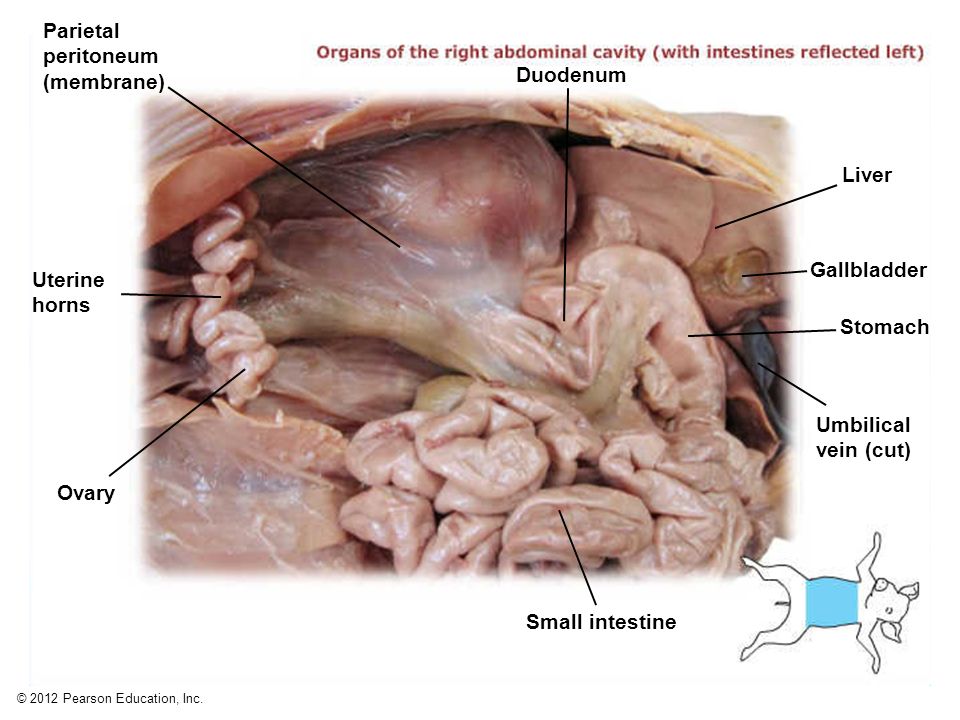The image is a detailed anatomical diagram displaying the organs of a pig's right abdominal cavity, with the intestines reflected to the left. A real picture of the pig's internal organs is shown, featuring various shades of grey, brown, and pink with a white film partially covering the upper left section. Each organ is clearly labeled with black lines connecting to specific sections. The highlighted organs include the duodenum, liver, gallbladder, stomach, umbilical vein (cut), small intestine, ovary, uterine horns, and the parietal peritoneum membrane. The labels use precise scientific terminology, with "duodenum" (D-U-O-D-E-N-U-M) and "parietal peritoneum membrane" (P-A-R-I-E-T-A-L-P-E-R-I-T-O-N-E-U-M) highlighted. The top right corner of the image features red text stating "organs of the right abdominal cavity (with intestines reflected left)." In the bottom right corner, there is a small illustration of a pig lying down with a blue-highlighted abdominal area, indicating the digestive system's focus. Additionally, the bottom left corner has a copyright mark indicating "2012 Pearson Education Incorporated."